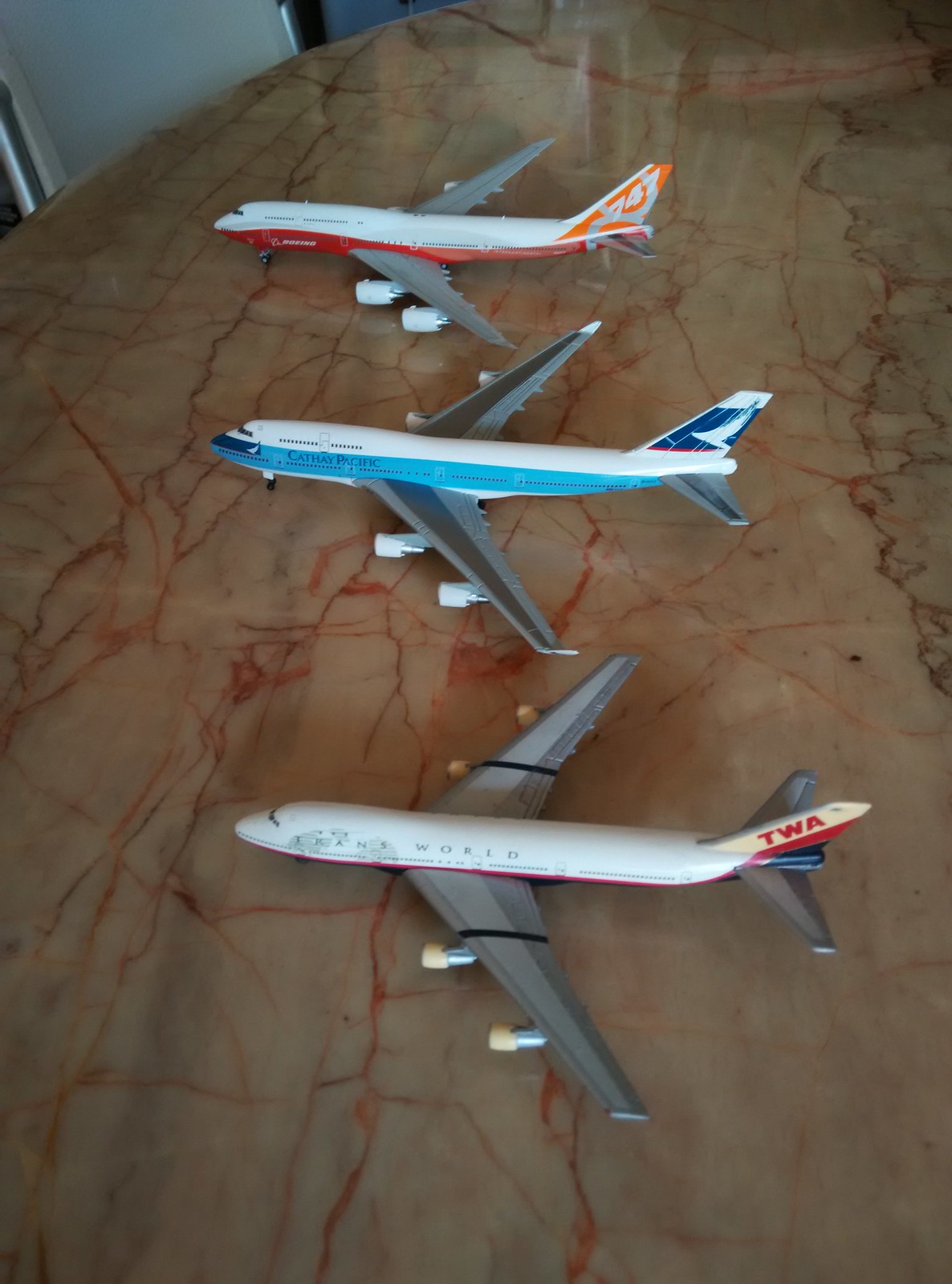In a dimly lit interior shot, a photograph captures three small model airplanes meticulously lined up on a marble table with striking dark red and orange marbling patterns. The vertically rectangular frame showcases the planes from bottom to top, each facing the left side of the frame. The planes sit on the reflective surface of the table, which adds a slight sheen and depth to the image.

The nearest plane to the camera is predominantly white with silver wings. Notably, its tail wing features red letters spelling out "TWA" alongside pale yellow and red coloring. The middle plane is characterized by a white top and a pale blue stripe running along its body, complemented by silver wings with a darker silver section in the middle. The furthest plane in the lineup has a white body with a dark orange stripe along the lower portion and "747" marked on its tail; this plane also features silver wings and an orange-colored section underneath the white body.

The subtle lighting and reflective surface emphasize the sleek design of these miniature models, making the marbling of the table and the painted details on each plane stand out vividly.